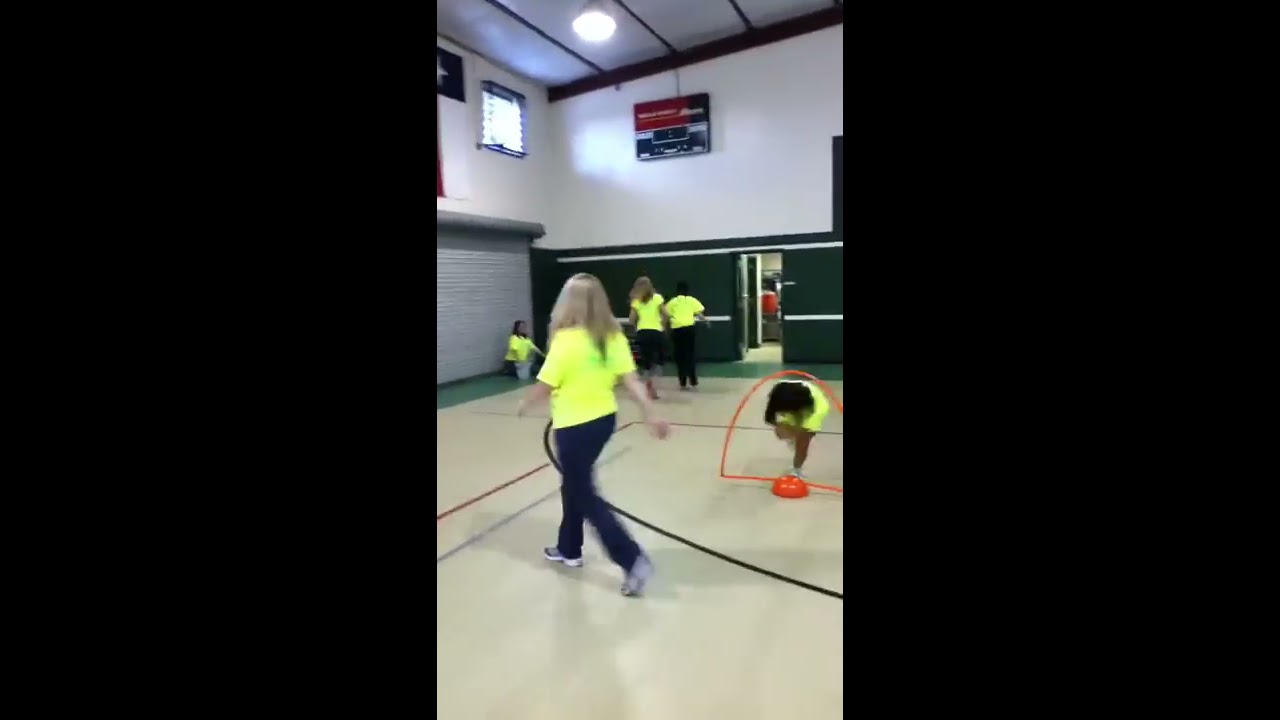The image captures an indoor gymnasium, partitioned into three sections with the left and right thirds displaying a thick black border. The center section reveals a detailed, albeit slightly blurry, view of the gym’s corner. The top half of the left wall is white, featuring a high-up window and a light source that casts a glare. The bottom half of this wall is gray, while the adjacent wall to the right is similarly white on the top half but green on the bottom, hosting what appears to be either a large scoreboard or an advertisement. Below, the court floor is light beige with markings, possibly blue or green around the edges.

Within the center of the scene, there are five women dressed in fluorescent yellow T-shirts, black pants, and sneakers, predominantly facing away. One woman on the right is bending down, seemingly reaching for an orange or red object, potentially a hoop. Additionally, there is a row of black metal doors along the wall, with one door noticeably open. The ceiling, painted white, includes a central, round light fixture contributing to the overall brightness of the room.